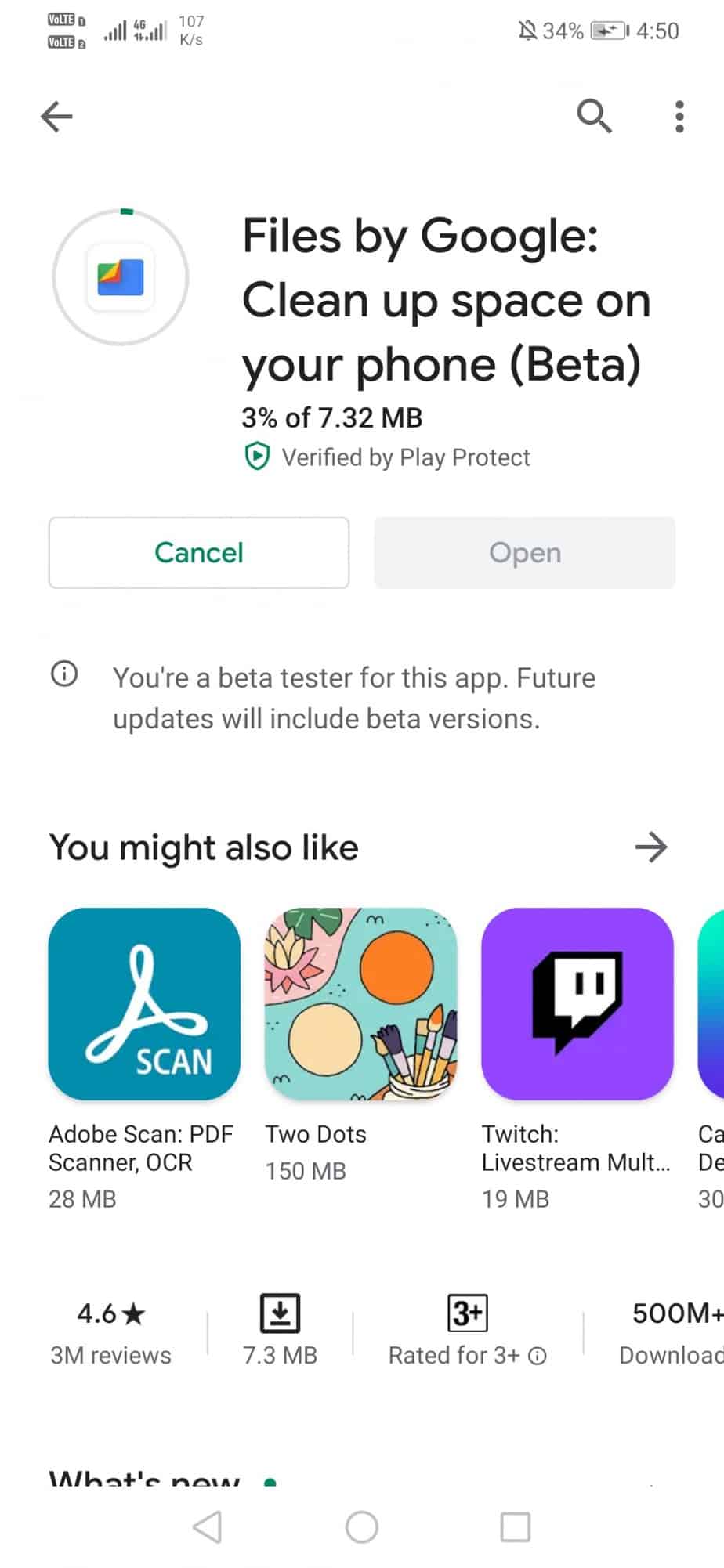A smartphone screenshot features various details about the Google Play Store. Visible on the screen are the signal bars indicating full cellular reception and a battery level at 34%. 

The time displayed is 4:50, and the user appears to be browsing for apps on the Google Play Store. Several navigation buttons are noticeable at the top, including a back button, a search icon, and a menu icon consisting of three vertical dots.

The user is on a page for the app "Files by Google," which offers to clean up space on the phone. This app is in its beta version, occupying 7.32 megabytes, and shows a status bar indicating that only 3% has been downloaded. The download is verified by Play Protect. The app icon is a multi-colored square encircled within a gray circle with a small segment in green to showcase the download progress.

Below the status bar, there are two buttons: "Cancel" in white font on a green background and "Open" in gray font on a gray background. The page includes a message stating the user is a beta tester and will receive future beta versions of updates.

In the "You might also like" section, there are three suggested apps: 

1. Adobe Scan: PDF Scanner, OCR, sized at 28 megabytes.
2. Twitch: Live Stream, with the size partially visible, indicating 19 megabytes.
3. An app with only a partially visible name, showing "CA" and "DE" on two lines, sized at 30 megabytes.

Additionally, there's a general ratings summary showing the app has 4.6 stars, based on 3 million reviews.